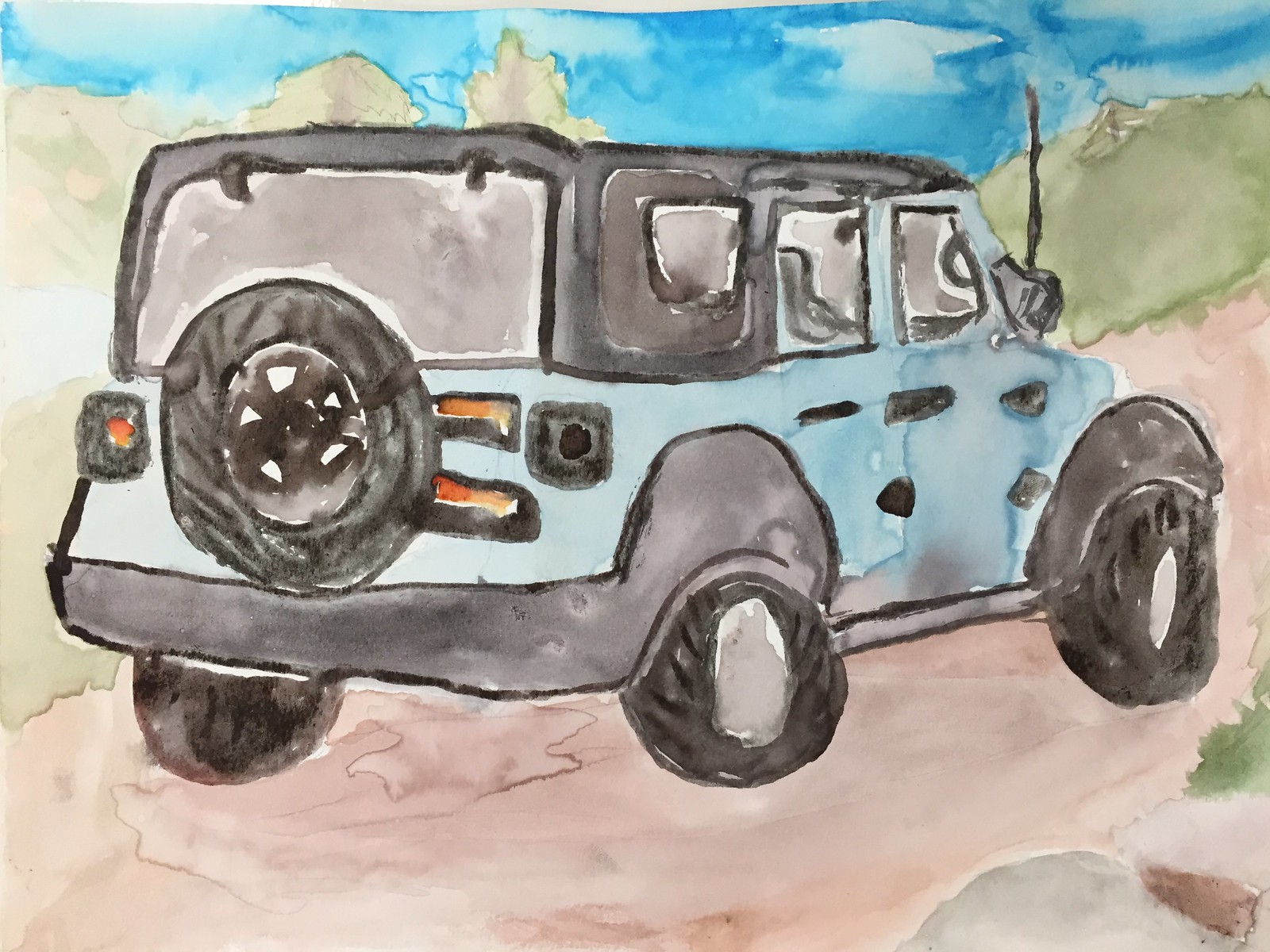A detailed watercolor painting depicts a blue jeep on a dirt road. The jeep, angled slightly away from the viewer, has its rear facing the left side of the picture while its front is directed towards the right. The vehicle features a black top and a black spare tire mounted on its backside. The passenger side of the jeep is visible, showcasing its sturdy build. The jeep is situated on a brown, earthy roadway, suggesting it's navigating a rugged trail. In the background, patches of green grass are visible in the upper right-hand corner, beneath a soft, serene sky that crowns the composition.